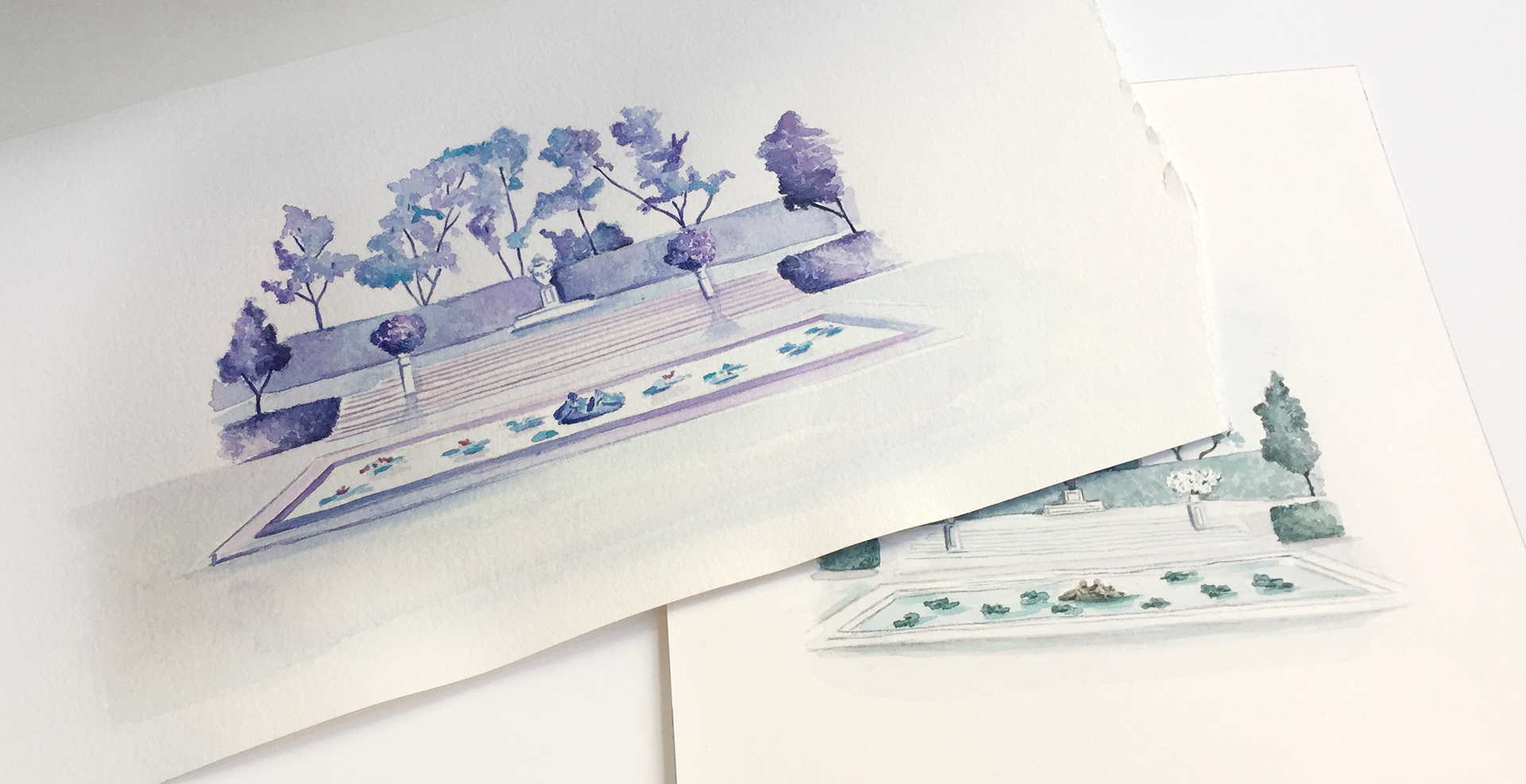Two pieces of notebook paper feature watercolor drawings of a well-landscaped garden courtyard. The papers appear to have been torn from a larger pad. Each drawing depicts a similar garden scene but uses different color themes: one primarily in shades of blue and the other in shades of green. The illustrations showcase a rectangular pond with lily pads at the forefront. Behind the pond is a staircase with about five or six steps, bordered by planters with bushes. Flanking the stairs are two trees, and additional trees along with large bushes, possibly a fountain or statue, fill the background. The overall design evokes a meticulously curated garden, reminiscent of a luxurious palace courtyard, like the one seen in Aladdin.